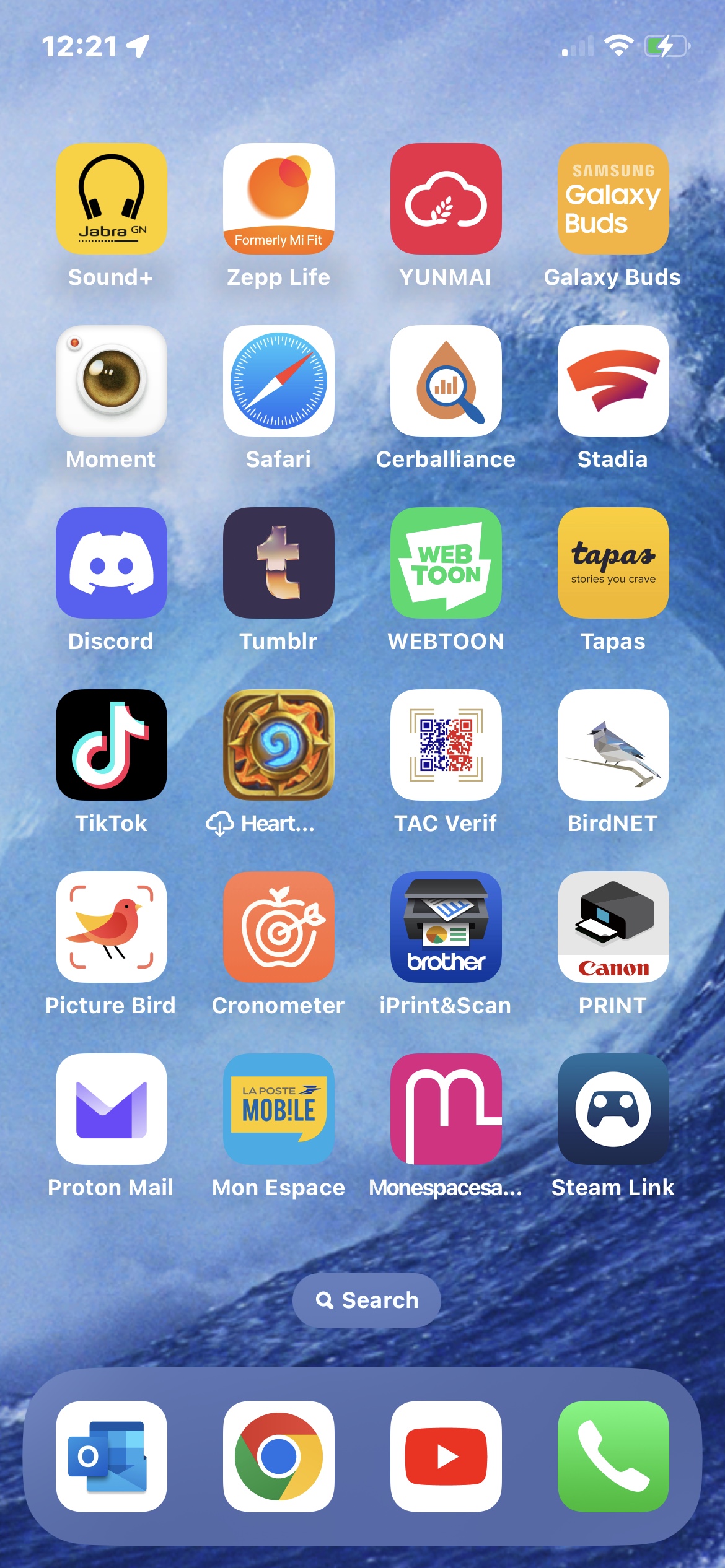This detailed caption describes a smartphone's home screen with various elements:

---

The image captures a smartphone's home screen at exactly 12:21 PM. The background showcases a dynamic blue design reminiscent of ocean waves, evoking the imagery of surfing. 

In the top-right corner, the status bar displays vital information:
- Wi-Fi connection at full strength
- A green battery icon indicating a 50% charge
- Signal bars with only the first bar, the smallest, highlighted in white.

Beneath the status bar, multiple rows feature an assortment of apps. The first row includes:
- Jabra Sound+
- ZeppLife
- UniMy with a distinctive red-and-white logo
- Samsung Galaxy Buds

The second row presents more apps:
- Moment, identified by a camera icon
- Safari, represented by a compass icon
- Serbalions
- Stadia
- Discord, featuring a cheerful white face on a purple background

Further rows continue with additional apps:
- Tumblr, marked with a lowercase "t"
- Webtoon, showcasing its logo on a white background with green text
- Tapas, with a yellow background and tagline "Stories you crave"
- TikTok with its recognizable symbol

Additional notable apps include:
- Heart Something (partially captured)
- Tac Verit
- BirdNet, denoted by a bird illustration
- Chronometer
- iPrint & Scan Brother
- Canon Print
- Proton Mail
- La Post Mobile
- Monescape (partially captured as Monospace)
- Steam Link

Below these, a search button is present, and just beneath it, four frequently used apps:
- YouTube
- WhatsApp
- Google Chrome
- A Microsoft app

This detailed home screen array offers insight into the diverse app usage and aesthetic preferences of the phone's owner.